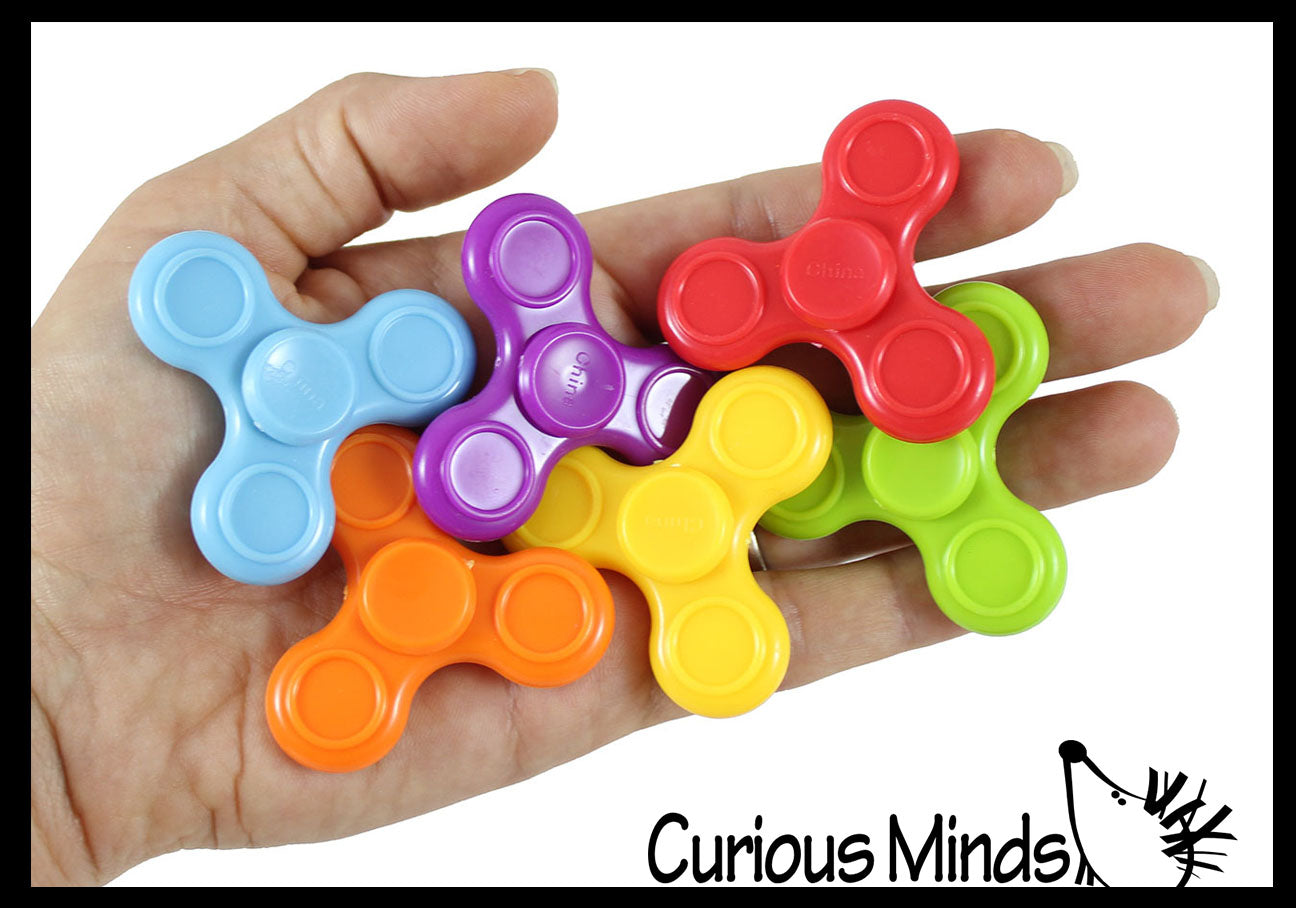In the image, a left hand with slightly long fingernails, palm up, holds six small, colorful fidget spinners. The hand enters the frame from the bottom left corner with the thumb pointing towards the top right. The fidget spinners are arranged with varying positions: some entirely on the palm, others partly on the fingers. Their colors are light blue, purple, red, orange, yellow, and green. The whole scene is set against a completely white background with a thin black border. In the bottom right corner, there's text that reads "Curious Minds" in a black font with capitalized C and M. Accompanying the text is a simple drawing of a hedgehog-like creature, characterized by beady eyes, a round nose, and spikes, gazing upwards towards the hand.